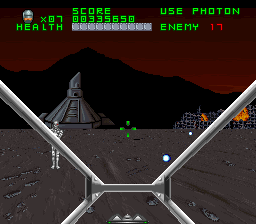In the top left corner of the image appears to be RoboCop, or possibly a character from Terminator. The interface section shows a time reading of '07', a health indicator, a score labeled '00335650', and two gray squares beneath. In the top right corner, it says 'Use Photon', with the enemy count at '17'. The central part of the image has multiple bars converging towards the center, intersected by horizontal bars, and below there are triangles forming a pattern. 

A robot is seen walking towards the screen on the left-hand side, with green crosshairs positioned in the center of the view. Blue orbs are situated on the right side. The background mainly features a dark, mountainous terrain with a red, shaded sky. There's a cone-like structure in the composition, and towards the middle-right, a jungle gym-like arrangement made up of numerous interconnected metal bars is visible. Two sections of the image illustrate structures engulfed in flames, giving the scene an intense, chaotic atmosphere.